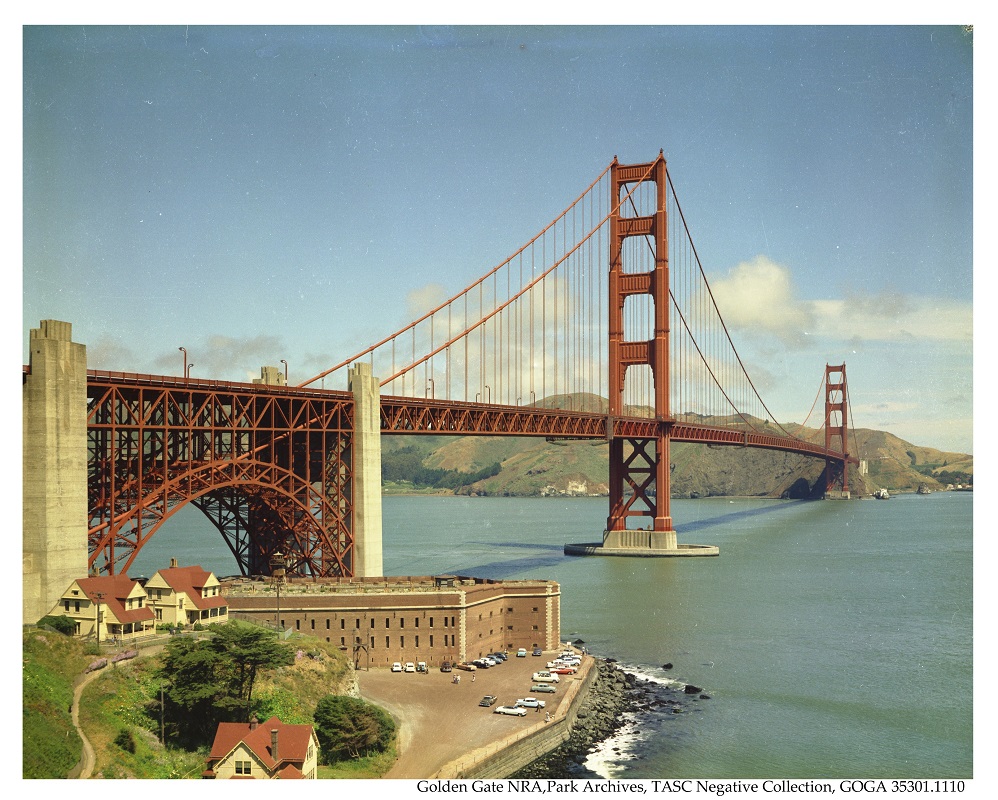A detailed and descriptive caption for the photo could be:

"This photograph showcases the iconic Golden Gate Bridge on a beautiful day with clear blue skies and a scattering of light clouds. The image, labeled 'Golden Gate NRA Park Archives TASC Negative Collection GOGA 35301.1110' in black text at the bottom, offers a breathtaking view from the side opposite Baker Beach, likely near Fort Point under the bridge. The signature red structure of the Golden Gate Bridge stands majestically against the calm waters of the bay, which reflect the sky and exhibit a subtle greenish hue with the bridge's shadow cast beneath. In the foreground, a parking lot edges towards the rocky shoreline, adjacent to a set of three yellowish buildings with reddish roofs. Two of these buildings are perched on a hill, accessible via a path and a small driveway, while the third sits alongside the road leading to the parking area. A few trees dot the scene, adding to the natural beauty. Tiny white flecks in the sky suggest this might be a scanned image. In the background, the distant hills and potential waterfront developments are faintly visible, completing this serene and picturesque landscape."